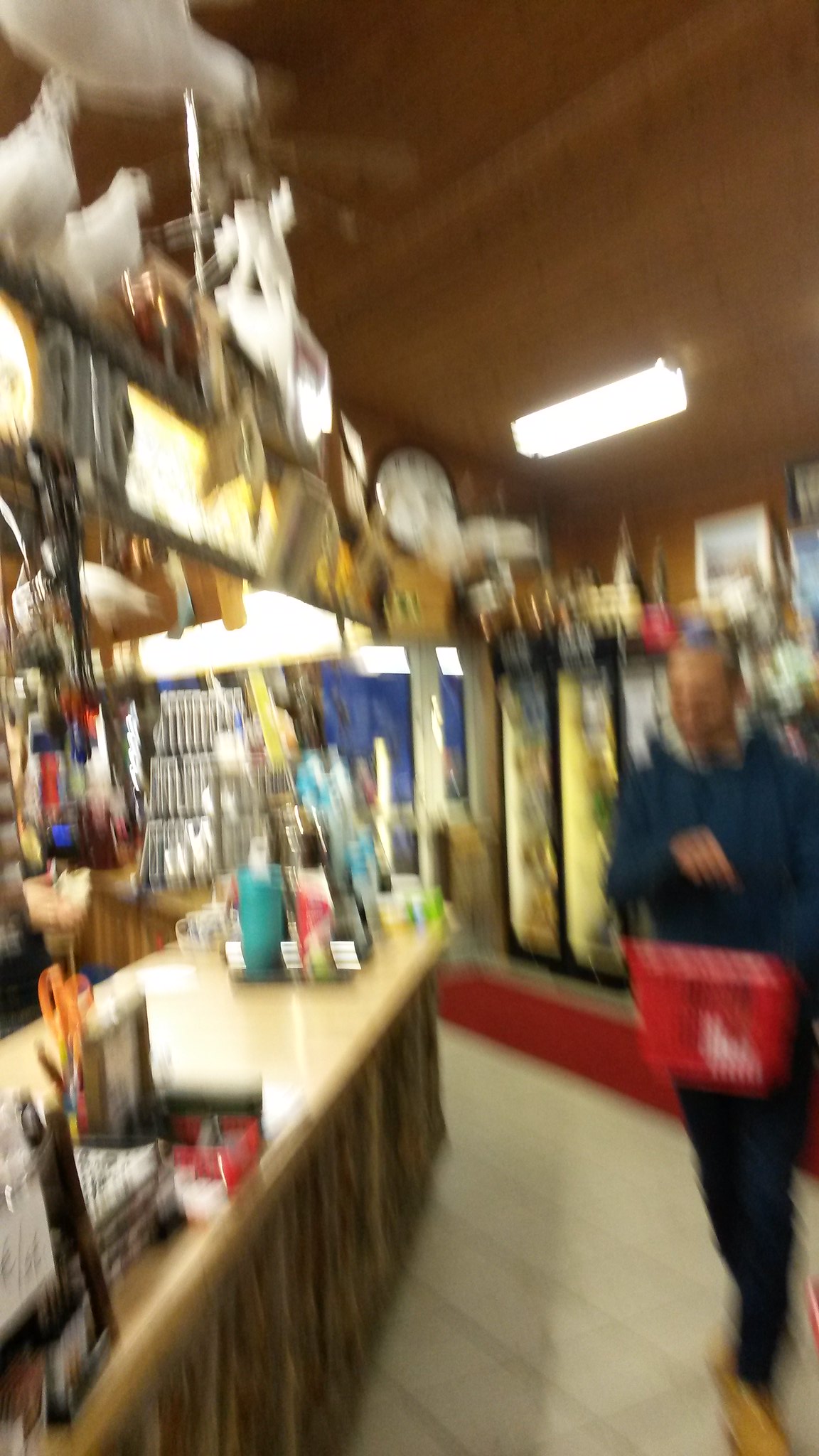The image depicts a blurred interior of a small, rustic store, perhaps a local mom-and-pop general store. The scene shows a man dressed in a dark top, likely black or blue, and black pants, carrying a red plastic shopping basket as he approaches a light brown wooden countertop with a darker brown front. The countertop is cluttered with office supplies and various impulse buy items, though they are difficult to discern due to the blurriness. Overhead, a drop-down ceiling is seen with multiple pieces of taxidermy, including birds and a European mount of a deer skull. On the right side of the image, illuminated coolers with clear glass doors and black frames, likely containing drinks or ice cream, add to the store's ambiance. The flooring is white tile, and fluorescent lighting bathes the scene in a bright, if not harsh, illumination. The overall setting combines rustic charm with everyday practicalities, though much of it remains obscured by the blur.